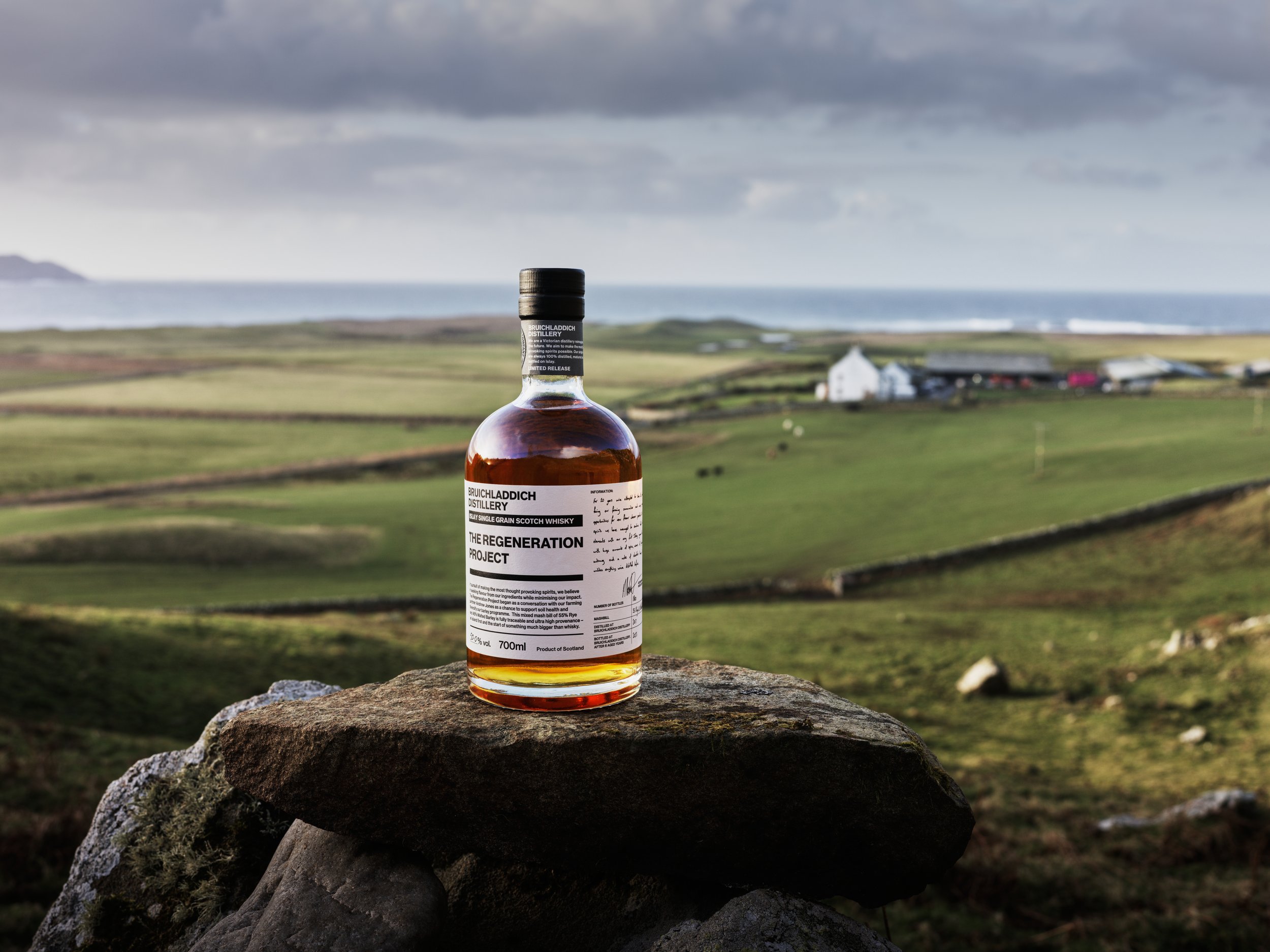A short, wide glass bottle of Single Grain Scotch Whisky labeled "The Regeneration Project" rests on an old granite rock. The whisky, with its transparent amber-brown hue, contrasts against the bottle's black cap and label, which also reads "Sambucha Latich Distillery." The setting is a picturesque countryside, featuring expansive green fields and farmland under a stormy, grey sky, suggesting imminent rain. In the distant background, there's a white farmhouse with a steel roof alongside a larger brown barn, and some cattle can also be seen grazing.